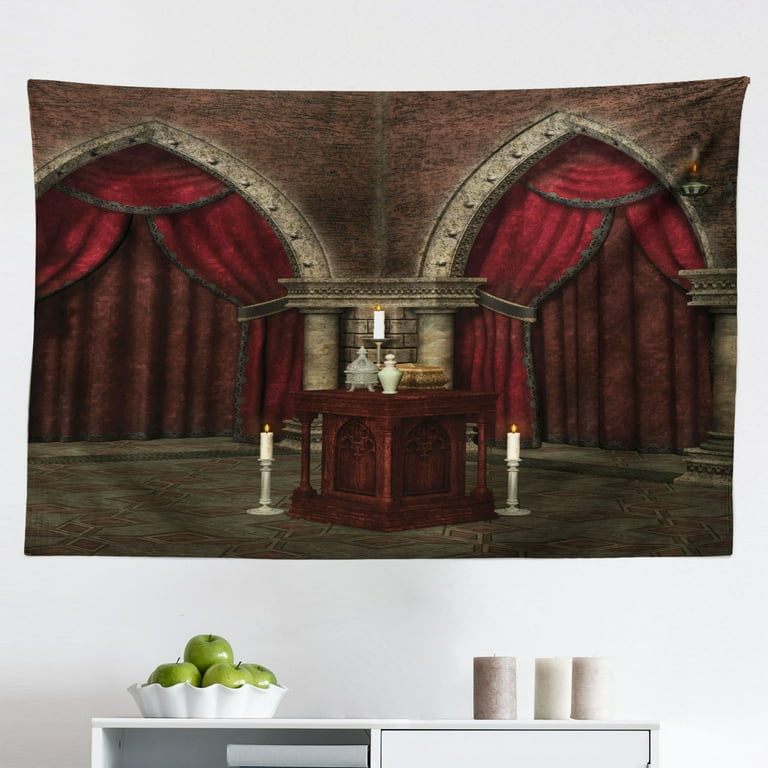In a room with an off-white wall, a fabric tapestry depicting a medieval castle interior hangs prominently. The tapestry showcases a majestic Gothic room with thick red curtains, exposed brick walls, and a tile floor. At the center, a dark brown altar table adorned with intricate royal designs holds candle holders with white candles, flanked by more candle stands on the floor. The scene features grand arched doorways with red and brown curtains, golden brown pillars, and a decorative fireplace, creating an opulent medieval atmosphere. Below the tapestry, a modern minimalist white table with a drawer and shelf is positioned, holding three cylindrical scented candles and a white bowl filled with green apples, bridging the historical and contemporary elements in the room.